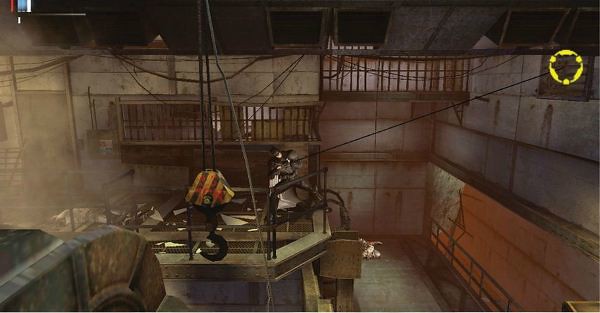Screenshot of a video game showcasing an industrial-themed level. The horizontal image features a gray, metallic ambiance characteristic of an old factory or warehouse. Dominating the center of the frame is a black object resembling a grappling hook, suspended by a black rope or line that extends across the scene. In the top right corner, a yellow circular dial with notches is prominently displayed, possibly indicating a game's mechanism or status. The top left corner houses a small blue object, though its identity is unclear due to its size. A gray vent occupies the bottom left of the image, adding to the industrial vibe, while the bottom right corner features a brown element affixed to the wall, contributing to the detailed environment. In the middle, gray bars add to the intricacy and immersive setting of what may be a mobile game or a stage within a larger video game.